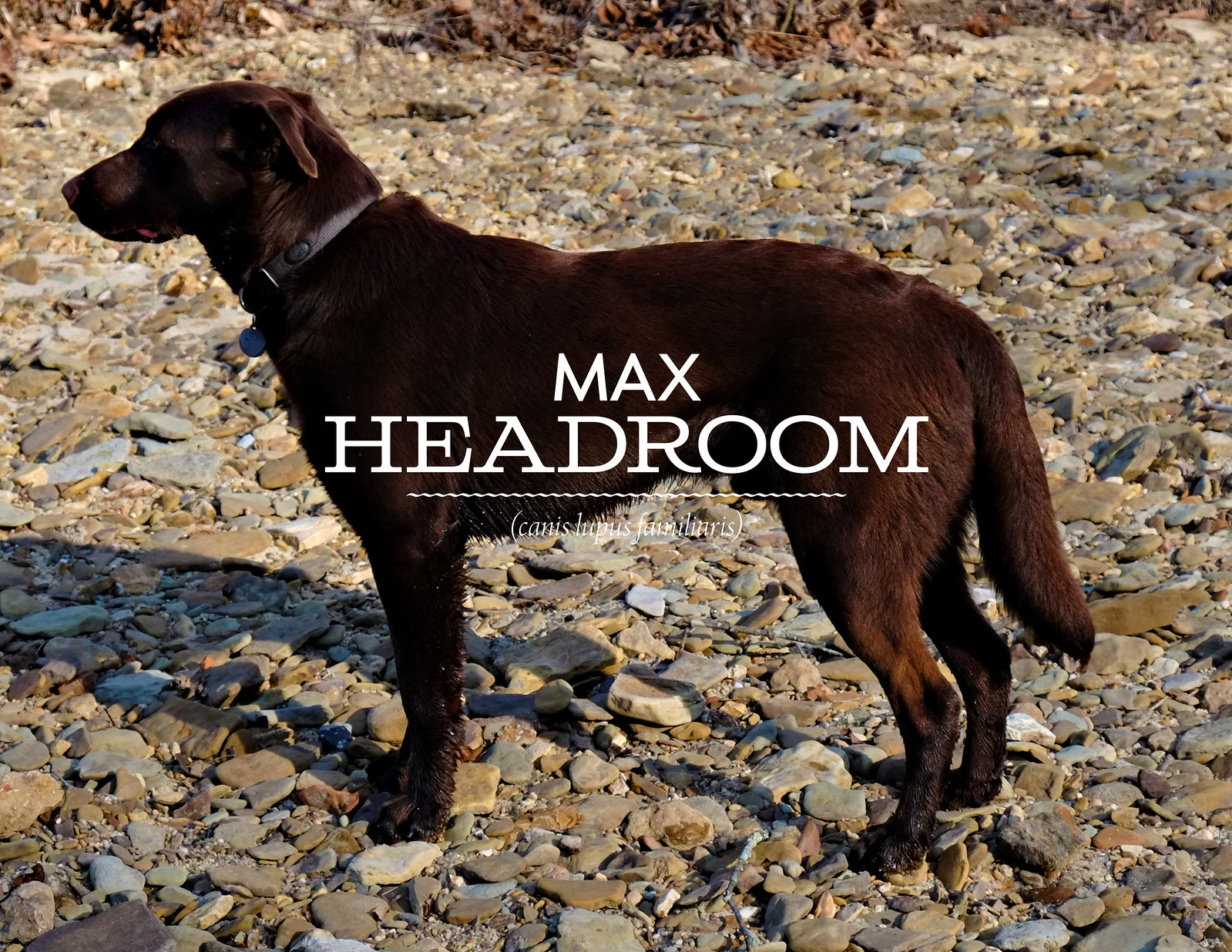This outdoor photograph captures a relatively large, chocolatey-brown dog with a serious and dedicated expression, looking toward the left. The dog stands with all four paws on the ground, which appear wet, suggesting a recent encounter with water. He's wearing a black or bluish-gray collar. The ground beneath him is a flat, rocky terrain, resembling the bottom of a dry lake or river bed, filled with pebbles and larger rocks. In the top part of the image, there's some foliage consisting of leaves and sticks, indicating it's late afternoon, with shadows clearly visible to the lower left of the dog. Overlaying the dog's body, the center of the image features a watermark that reads "Max Headroom." Below this, separated by a curved line, is the Latin text "Canis Lupus Familiaris," denoting the species of the dog.